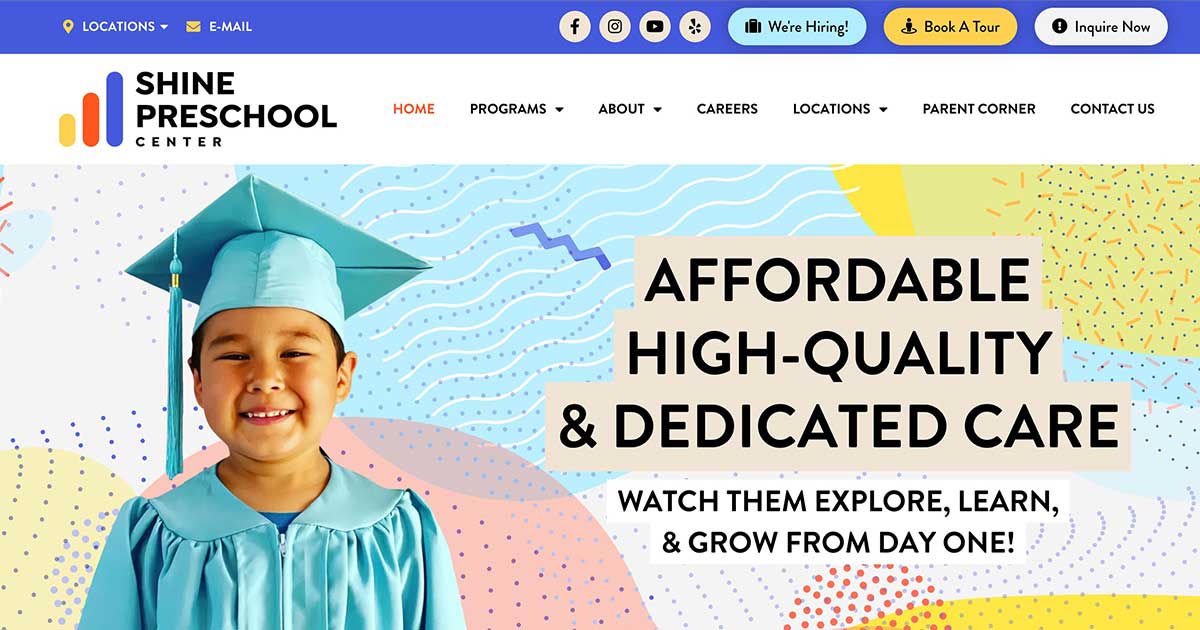This image showcases the homepage of Shine Preschool Center's website or app interface, highlighting its well-organized and visually appealing design. At the top of the page, there is a distinctive blue navigation bar featuring options such as "Locations," "Email," and various social media icons for platforms like Facebook and Instagram. Additionally, there are buttons labeled "We're hiring," "Book a tour," and "Inquire more." Below the bar, the Shine Preschool Center logo is prominently displayed.

The header also includes a menu with links to "Home," "Programs," "About," "Careers," "Locations," "Parent Corner," and "Contact Us." The main focus of the page is a vibrant image of a smiling child dressed in a turquoise graduation gown, symbolizing achievement and celebration. To the right of the child, a tagline reads, "Affordable, High Quality, and Dedicated Care. Watch them explore, learn, and grow from day one."

The background is decorated with playful and colorful designs, including yellow, red, and blue circles, as well as dotted circular patterns, adding a lively and inviting touch to the page. Overall, the website’s layout is sleek, well-designed, and easy to navigate, making it an attractive option for parents considering Shine Preschool Center for their children's early education.